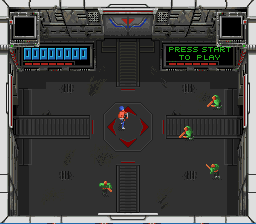The image depicts a top-down view of a third-person video game set in a futuristic military base that appears to also serve as a computer database room. The room is a square with dark gray, metal-like floors that feature what seem to be vents, and light gray, metallic walls. There are four exits or entrances situated on each side of the room that are grey. In the center of the room is a circular area surrounded by four directional arrows. The main character, positioned in this central area, is topless and wears blue pants, white sneakers, and a blue hat. This character contrasts with the four enemies or opposing team members, who are dressed in green outfits with black pants, white shoes, and each carrying orange weapons or wooden bats. Additionally, there are red triangles pointing towards the center stage from each directional area, hinting at a strategic combat zone. The top right corner of the screen displays "Press Start to Play" in green text on a black computer screen, with red lines underneath, while the top left corner shows a score of zero against a backdrop of blue rectangles.